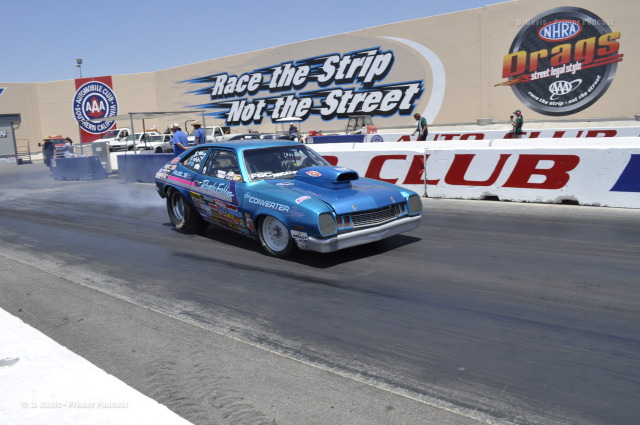The image captures a vibrant and dynamic scene of a blue drag race car, identified as a Pinto, poised on a drag strip. The car is adorned with numerous decals and logos, including notable ones such as NHRA Drags and Triple-A. Behind the car, the drag strip wall displays the message "Race the Strip, Not the Street" in white lettering outlined in black, with a backdrop of blue flashes enhancing the racing theme. The wall also features other inscriptions such as "Automobile Club Southern California" and "Street Legal Style." The scene is bright and clear, set outdoors during the daytime under a blue sky. The car appears to be revving up at the starting line, with smoke billowing from its tires, suggesting imminent acceleration. In the background, various vehicles and a few people are visible, adding to the lively atmosphere of the race event. Additionally, a watermark reading "D Davis Printer Primer Podcast" is subtly placed in the bottom left corner of the photo.